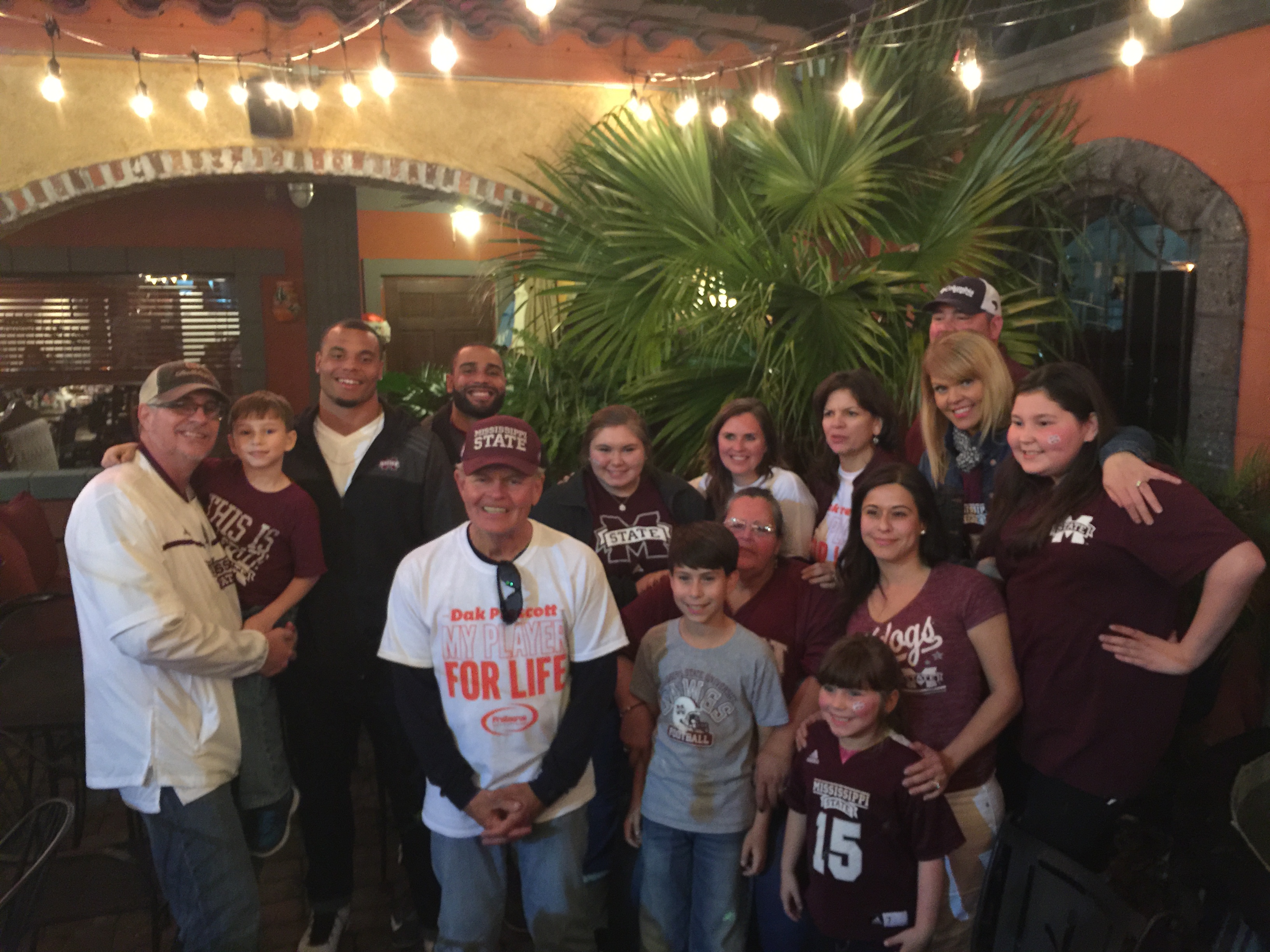In this festive and lively photograph taken in what appears to be a Mexican-style restaurant, a diverse group of around 15 people is gathered for what seems to be a family or team celebration, possibly a benefit event. The restaurant setting features arched doorways and windows, string lights, and a large palm tree in the corner, creating a welcoming atmosphere. Most of the group members are wearing burgundy shirts emblazoned with "Mississippi State" and various team or player numbers, including a notable long-sleeved shirt dedicated to "Dak Prescott, my player for life." 

Prominently in the foreground, an elderly man in a maroon Mississippi State cap is seen holding a young child. Next to him, a man with glasses and a cap, dressed in a white shirt, also holds a boy. The group consists predominantly of Caucasian individuals, with a mix of women, men, and children, including both young girls and boys, varying in age from young children to middle-aged adults. Additionally, there are two well-built men of African descent dressed in dark tracksuits standing directly behind the elderly man.

The photograph captures a moment of joy and camaraderie, with everyone smiling and enjoying their time together in this cozy and cheerful setting.